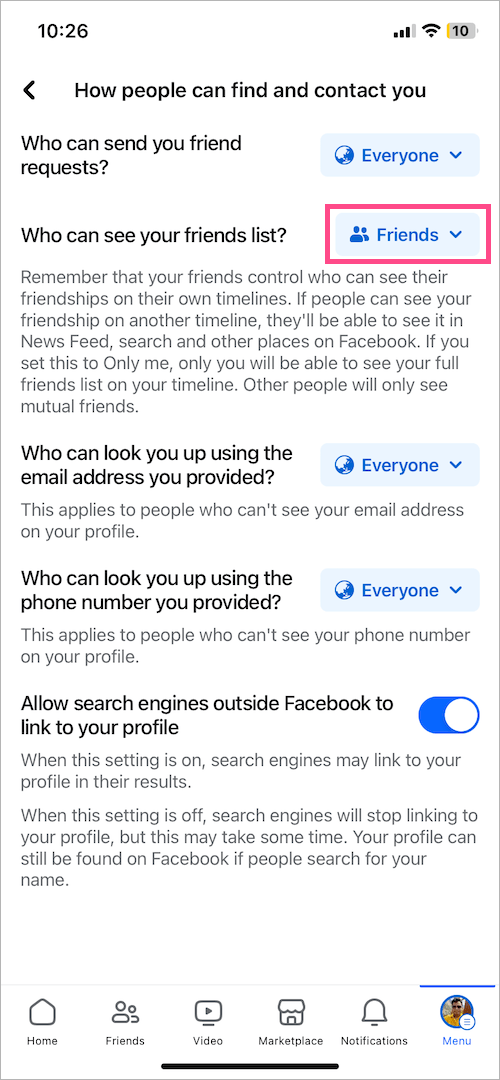The image is a screenshot taken on a cell phone, displaying specific privacy settings on a Facebook profile. In the top left corner, the time is shown as 10:26, while the battery icon at the top right indicates a 10% charge.

The central focus of the screenshot is a section of the privacy settings, outlined by a red rectangle. The settings detail various options for user visibility and contact permissions:

1. **Who can send you friend requests?** Everyone.
2. **Who can see your friends list?** Friends.
   - A note emphasizes that your friends control who can see their friendships on their own timelines. If your friendship appears on another timeline, it will be visible in newsfeeds, search, and other areas on Facebook. Setting this to "Only me" allows only you to see your full friends list on your timeline, while others will only see mutual friends.
3. **Who can look you up using the email address you provided?** Everyone.
   - This applies to those who cannot see your email address on your profile.
4. **Who can look you up using the phone number you provided?** Everyone.
   - Similar to the email setting, this applies to users who cannot see your phone number on your profile.
5. **Allow search engines outside Facebook to link to your profile:** The slider button is set to "On."
   - When enabled, search engines may link to your profile in their search results. Disabling this setting will eventually stop search engines from linking to your profile, but this may take some time. Nevertheless, your profile can still be found on Facebook through direct name searches.

At the very bottom of the screenshot, there are navigation options labeled: Home, Friends, Video, Marketplace, Notifications, and Menu.